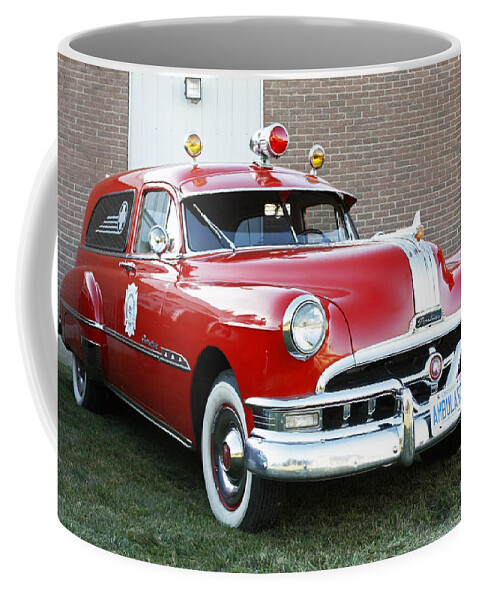This detailed up-close photo of a coffee cup features a vivid illustration wrapping around it. The central image showcases a classic 1950s-60s style emergency vehicle, likely a fire chief's car or an ambulance. This vintage car highlights a bright, fire truck red body with notable chrome accents, including a wide chrome strip adorning the center of its hood and chrome trim along the sides. Atop the vehicle are distinctive old-style flashing lights: a central red light flanked by two yellow lights, all housed in chrome. Over the split windshield with its upright wipers lies a metal visor. The car boasts white wall tires, complete with chromed hubs and a red accent at their centers. Additional details include a white star symbol on the side, an emblem resembling a police badge, and a somewhat blurry license plate on the front that appears to read "ambulance." Surrounding the vehicle is a background of gray brick with a thick white stripe, and rough grass below. This nostalgic scene is captivatingly captured in the print on the coffee cup.